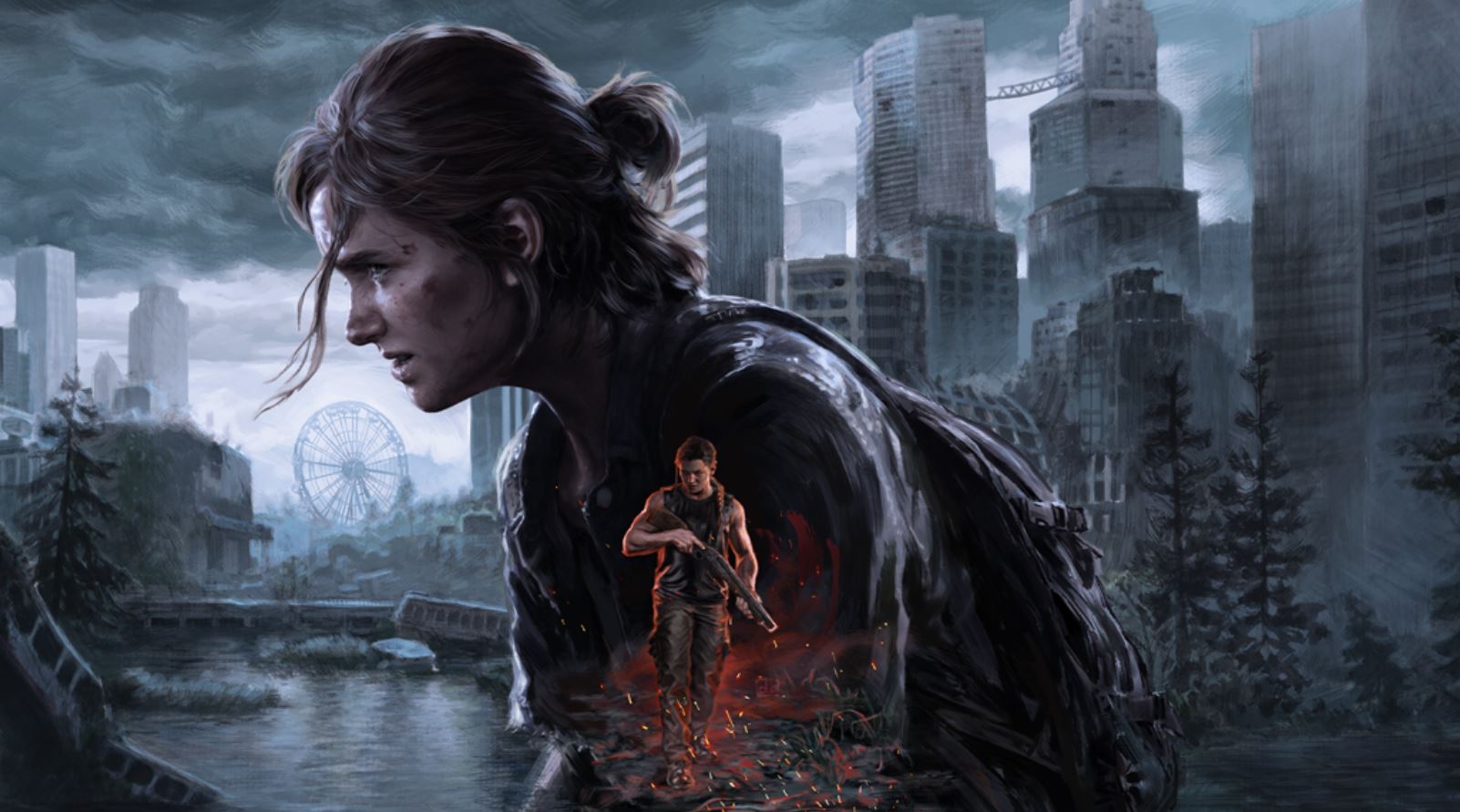In this detailed digital painting inspired by the video game "The Last of Us," the foreground features a young woman with dark brown hair tied up in a bun, although some hair falls loosely around her face. Her appearance is rugged and dirty, with visible dirt and signs of wear on her face and clothes, suggesting she has endured a long and harsh journey. She is dressed in a black jacket and black backpack, kneeling down amidst an apocalyptic urban landscape.

The city behind her is marked by dilapidated, decaying skyscrapers and buildings, with many broken windows, giving off a sense of abandonment and ruin. The dark and cloudy sky enhances the somber mood of the scene. On the right side of the image, lush green evergreen trees contrast starkly with the destroyed urban environment.

In the bottom left corner, there's a large lake or pond, adding an additional layer of depth to the scene. Nearby, a rusty, decaying Ferris wheel stands as a lonely sentinel among the ruins.

A striking feature of the painting is the male figure embedded within the central part of the woman's body, as if he represents an integral part of her. This man has short hair and is depicted walking towards the viewer, wearing a black sleeveless shirt and black pants. He carries a shotgun with a brown stock and appears to be trudging through fire or lava, with amber embers rising from the ground around his feet.

The overall color palette of the artwork is dominated by dark grays, blacks, and blues, with striking red accents centering around the man holding the gun. The painting vividly captures the grim and chaotic atmosphere of a world in the throes of an apocalypse.